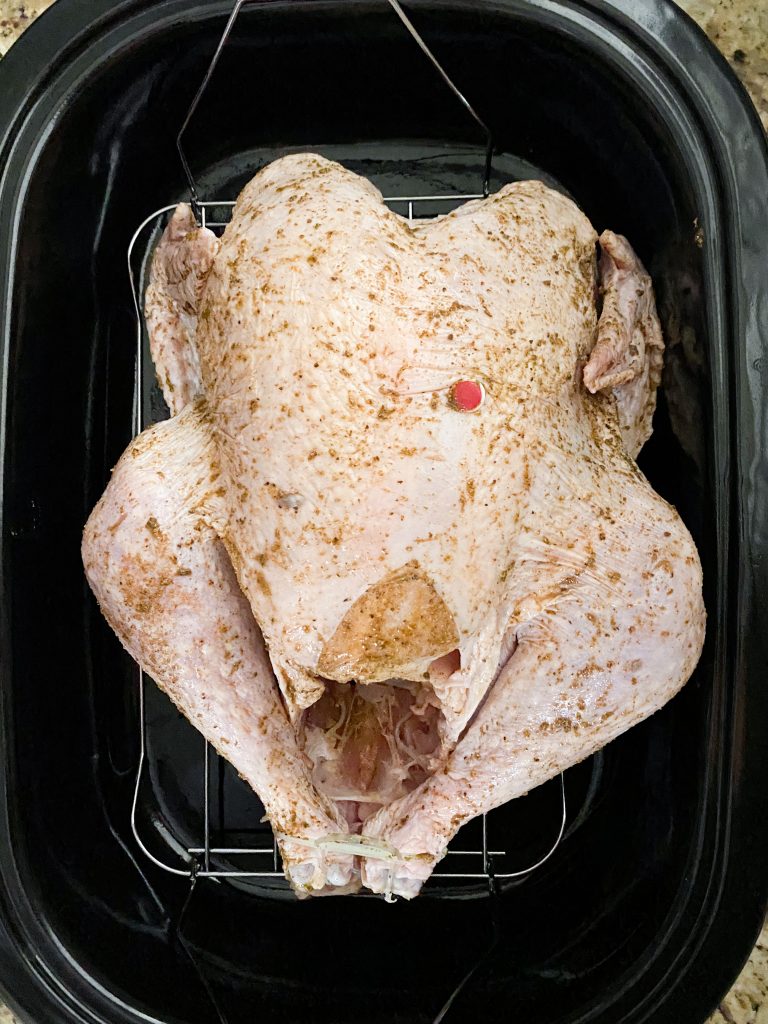The image shows a very close-up view of what appears to be a whole, raw turkey placed in a large black roasting dish, likely in preparation for baking. The turkey, which has its drumsticks bound together with twine, is positioned on a metal wire rack inside the roasting pan. The white skin of the turkey is generously slathered with a brown seasoning mixture, possibly containing brown sugar. Near the center of the turkey, there's a red-tipped temperature probe inserted, which will pop up when the bird is fully cooked. The roasting dish, positioned on a countertop or table, contrasts with the turkey's textured surface and the metal wire rack, setting the scene for an imminent cooking process.